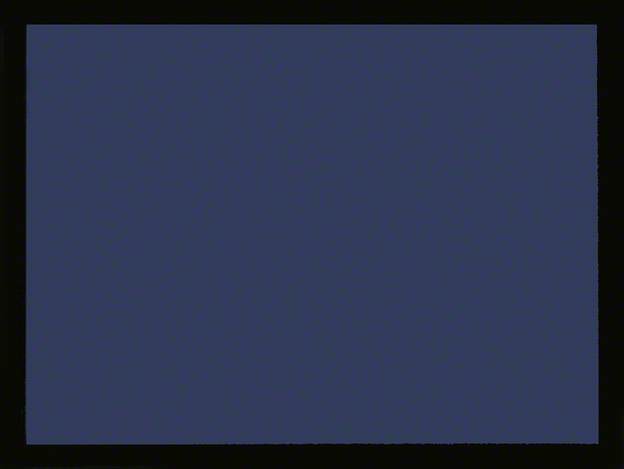The image is a minimalistic abstract rectangular piece, slightly wider than it is tall, framed by a thin, consistent black border. Dominating the central area is an expanse of dark bluish-gray or navy blue devoid of any text or distinct objects. The top section of this central area features some barely visible lighter blue lines running across. Surrounding the central blue expanse, particularly on the right and bottom edges, is a subtle, almost fuzzy gray material, with the left edge appearing blurrier and less defined. Overall, the image contains only two primary colors – the dark blue center and the narrow black border – leaving its exact nature as whether it is a painting or a digital creation, open to interpretation.